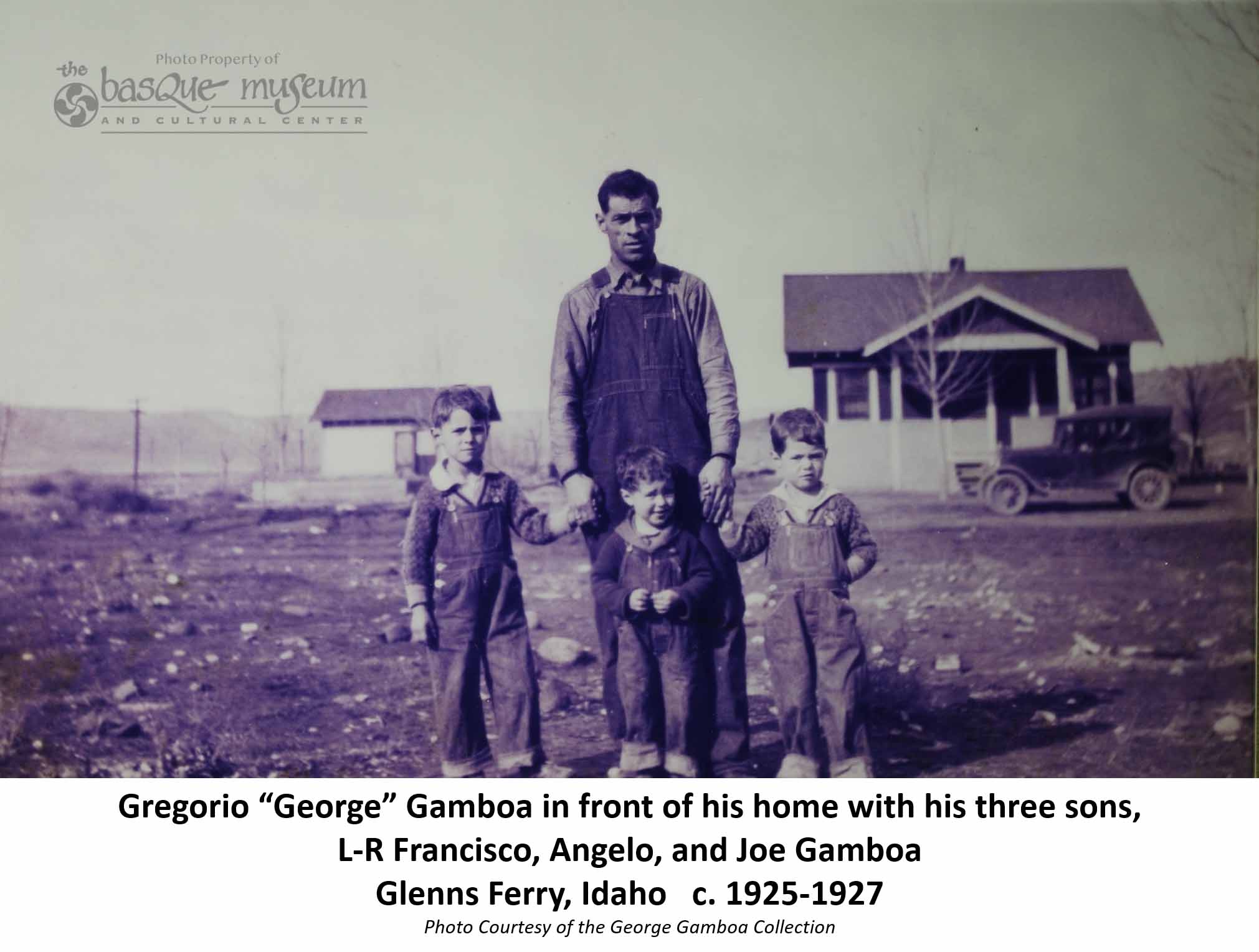This vintage black and white photograph, tinted with a faint bluish or darkish hue, captures Gregorio "George" Gamboa standing in a dirt field in front of his modest home in Glens Ferry, Idaho, with his three young sons, Francisco, Angelo, and Joe Gamboa, circa 1925-1927. George is dressed in a long-sleeved shirt and overalls, clasping hands with Francisco on his left and Joe on his right, while the youngest, Angelo, stands directly in front of him. All the boys are similarly attired in overalls over collared long-sleeved shirts. To their right, an old-style car is parked near the small house that resembles a shack, and next to it, a smaller storage building is visible. The top left corner of the photograph bears the inscription "Photo property of the Basque Museum and Cultural Center." The caption beneath the image reads, "Gregorio 'George' Gamboa in front of his home with his three sons, L-R: Francisco, Angelo, and Joe Gamboa, Glens Ferry, Idaho, circa 1925-1927. Photo courtesy of the George Gamboa collection." Rocks are scattered on the ground, and the sky appears overcast, enhancing the photograph's nostalgic atmosphere.